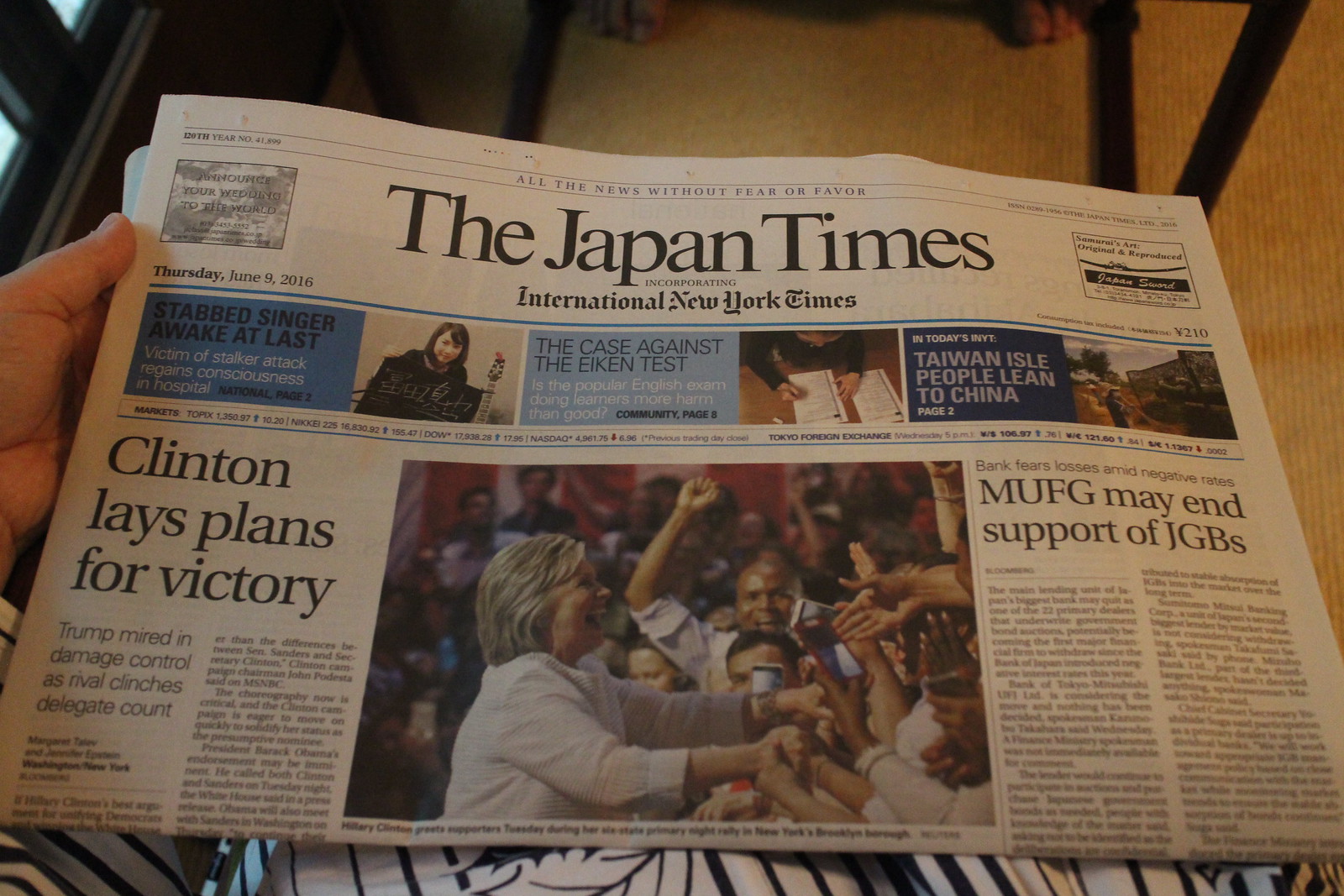In this detailed rectangular image, which has a postcard-like orientation with a longer width than length, a hand is visible in the bottom left corner grasping a copy of The Japan Times, which is associated with the International New York Times. The newspaper is dated Thursday, June 9, 2016. The prominent headline reads "Clinton lays plans for victory," accompanied by a photograph of Hillary Clinton greeting a cheering crowd of supporters during her presidential campaign. Directly beneath this headline, although not fully legible, there is a reference to Trump's "mired in damage control."

To the right, another headline reads "MUFG may end support for JGBs." Among the smaller stories included on the front page, one headline details "Stabbed singer awake at last; victim of stalker attack regains consciousness in hospital." Another story, situated centrally at the top, discusses "The case against the ICAN test," while to the right, it is mentioned that "Taiwan isle people lean to China."

The text is predominantly in English, despite the newspaper's Japan-oriented title, reflecting its international reach.